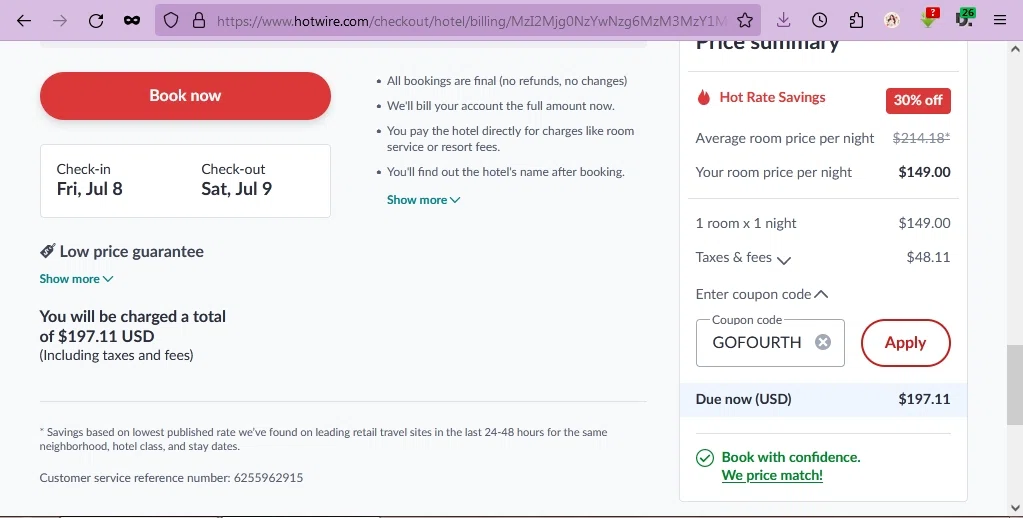This detailed screenshot captures the interface of Hotwire.com, a popular hotel booking website. At the top of the purple navigation bar and the search engine field, the site's URL is prominently displayed: "hotwire.com" in black letters.

A prominent red button labeled "Book Now" in white is a central call-to-action element. Below this, booking details are indicated: "Check-in Friday, July 8th, Check-out Saturday, July 9th," with a note about a "Low Price Guarantee." 

Adjacent to these details, a green "Show More" link with a downward arrow hints at additional information. The total cost, "$197.11 USD (including taxes and fees)," is prominently displayed.

Further down, a fine print section provides context about savings: "Savings based on the lowest published rate found on leading retail travel sites in the last 24 to 48 hours for the same neighborhood, hotel class, and stay dates," accompanied by a customer service reference number: 6255962915.

Four important booking conditions are listed with bullet points:
- "All bookings are final (no refunds, no changes)."
- "We'll bill your account the full amount now."
- "You'll pay the hotel directly for charges like room service or resort fees."
- "You'll find out the hotel's name after booking."

On the right, a "Price Summary" section provides a detailed cost breakdown:
- "Hot Rate Savings: 30% off" in red.
- A crossed-out "Average room price per night: $214.18" in black.
- The actual "Room price per night: $149" listed below.
- "One room, one night: $149."
- "Taxes and fees: $48.11" with an adjacent drop-down arrow.

An "Enter coupon code" field with a drop-down arrow pointing upwards currently displays the code "goforth," accompanied by an "Apply" button.

A final summary, "Due now (USD): $197.11," is followed by a green label, "Book with confidence," featuring a green checkmark. An underlined "Reprice Match" link is also provided for reassurance.

There is no further text in the image, confirming it as a screenshot from the Hotwire.com booking platform.